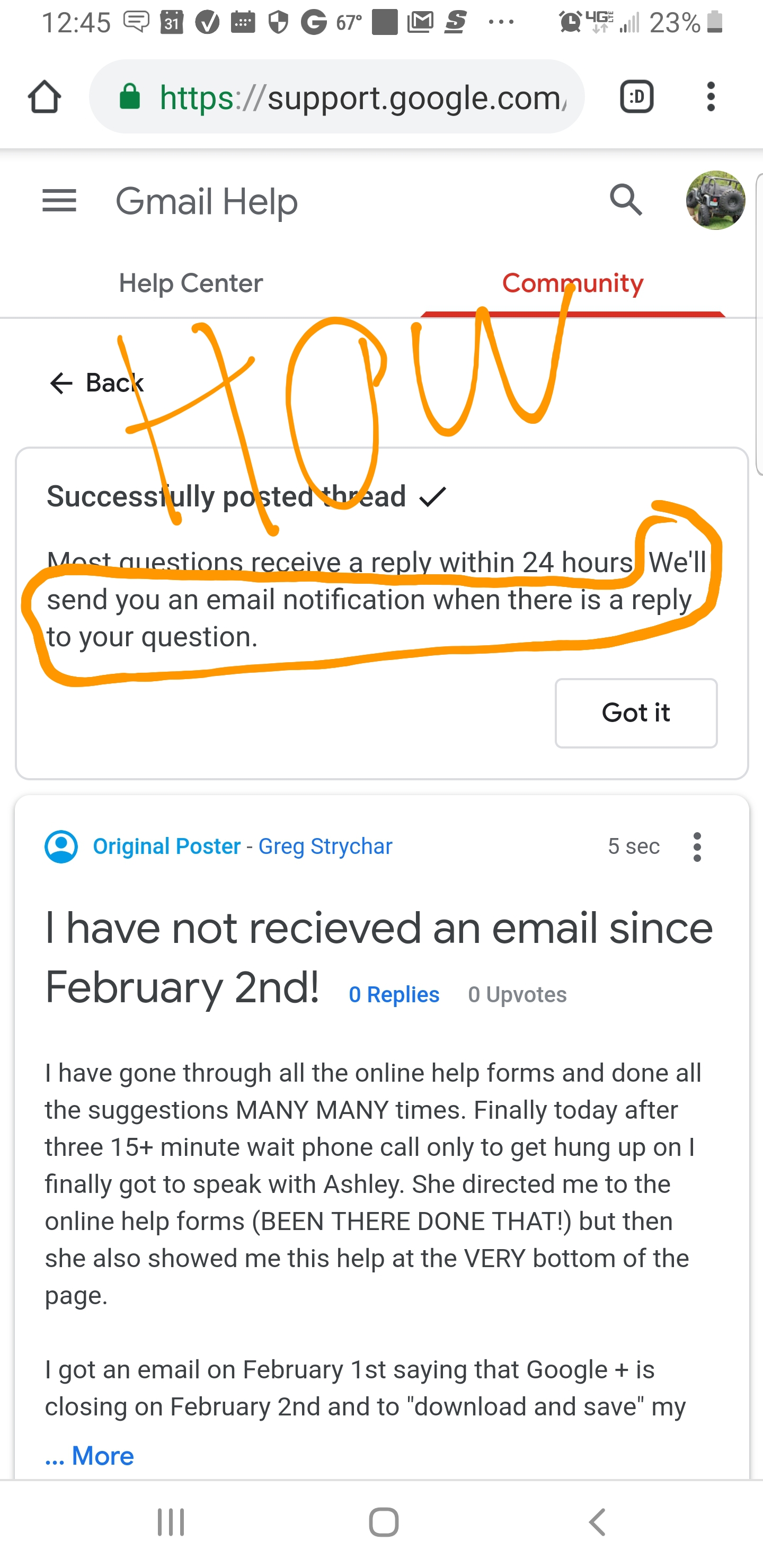This image is a detailed screenshot taken from a smartphone, displaying a webpage from support.google.com. At the top of the page, it clearly shows the header titled "Gmail Help." On the right side of the header, there is a magnifying glass icon, likely representing a search function, and an image that resembles a Jeep. 

Below the header, two options are presented: "Help Center" and "Community," with the "Community" option highlighted in red and underlined, indicating it is the current selection. On the left side of the screen, there is a "Back" button with a left-pointing arrow. 

The main body of the webpage includes a notification enclosed in a box, stating "Successfully posted thread" accompanied by a green checkmark. The notification further states, "Most questions receive a reply within 24 hours. We'll send you an email notification when there is a reply to your question," with the last sentence circled in orange and annotated with the comment "How about that" in matching orange text.

Below this, the original poster named Greg Stryker has shared his issue, exclaiming, "I have not received an email since February 2nd!" Greg elaborates that he has meticulously followed all online help suggestions numerous times. He recounts his frustrating experience of calling support thrice, enduring 15-minute waits each time, only to be hung up on. Eventually, he managed to speak with a support agent named Ashley, who redundantly directed him back to the online help forums he had already exhausted. However, Ashley pointed out some additional help resources at the bottom of the page. 

Greg's post includes an important note that he received an email on February 1st notifying him about the closure of Google Plus on February 2nd, instructing him to download and save his data. His full message trails off with an ellipsis followed by "more" in blue text, indicating additional content not visible in the screenshot.